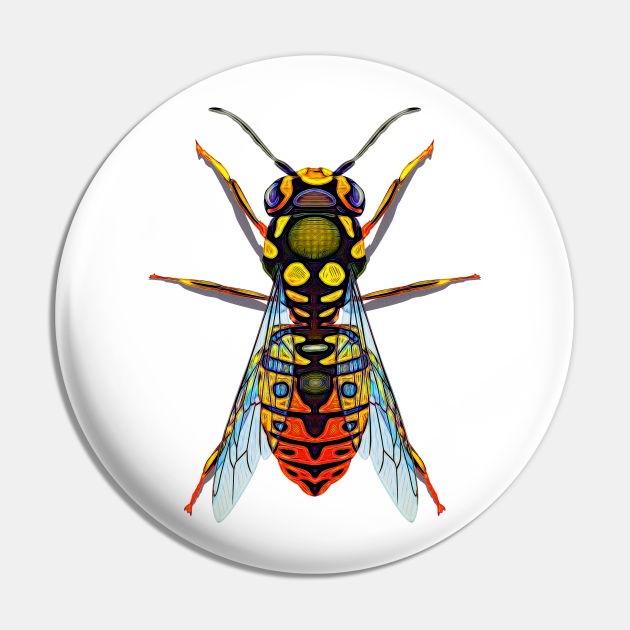The image features a drawn, highly stylized and colorful depiction of an insect, possibly a bee or hornet, viewed from above. The insect is set within a circular frame that has a predominantly white background with subtle gray around the edges. This circle is placed on a light gray, rectangular background. The insect's body includes a dark triangular thorax and an elongated, oval-shaped abdomen that narrows to a point. It has six legs, two extending from the center and four from the lower part of the body, all ending in red tips. The head is adorned with two antennae and has an eye on each side. The wings are thin, bluish, and exhibit visible veins. The whole composition is colorful and vibrant, with shades of blue and green accentuating the insect’s form. The details are crisp, making the overall image striking and visually engaging.